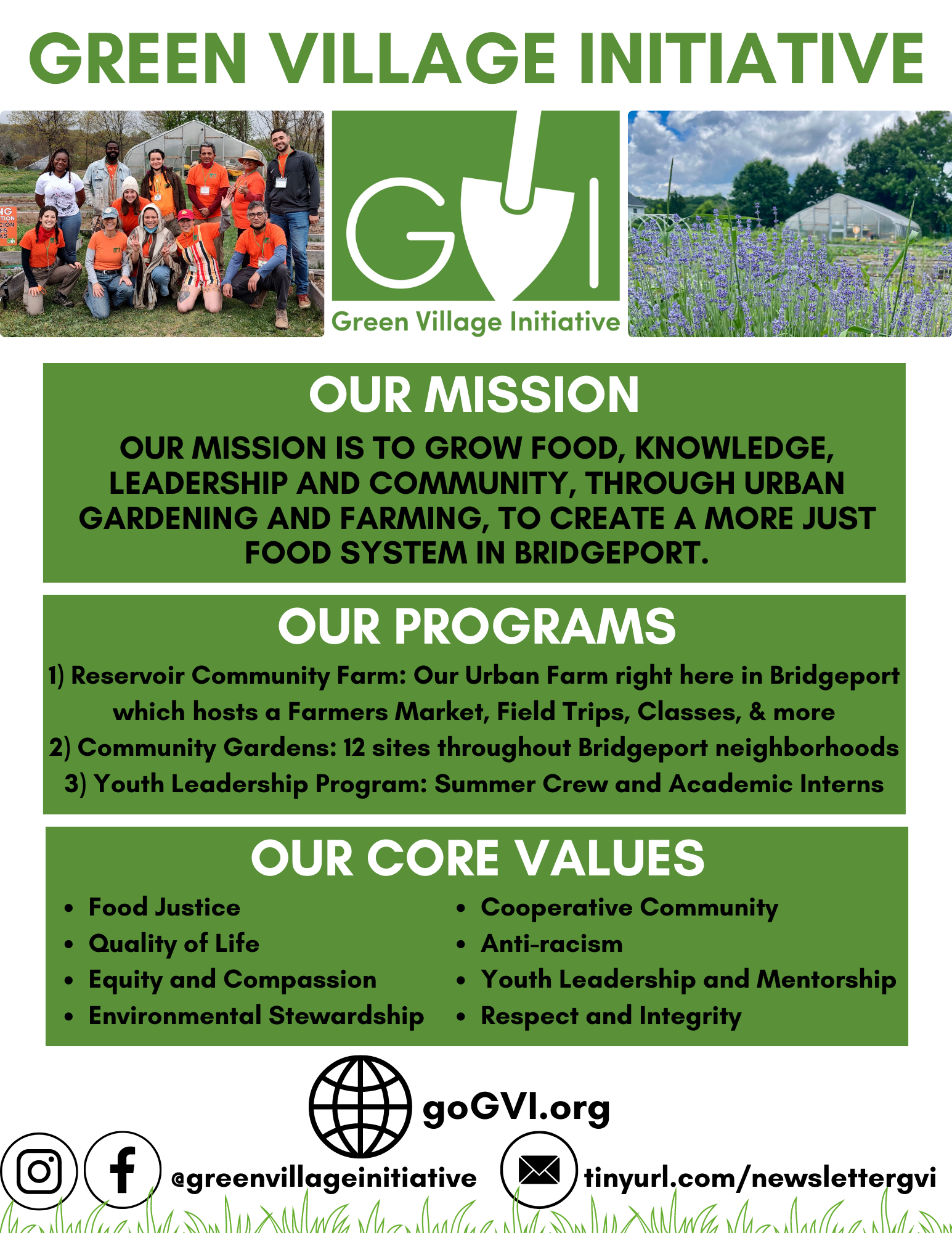The detailed poster for the Green Village Initiative features a vibrant green header displaying "Green Village Initiative" prominently. Below, it contains three distinct images and informative blocks. The first image on the left shows a group of people, mostly wearing orange t-shirts, posing outdoors with a backdrop of trees and a building, suggestive of a communal or mission-driven activity. The center image presents the initials "GVI" with the 'V' visually represented as a shovel, reinforcing the initiative's agricultural focus. The third image on the right depicts a greenhouse with a slender field of purple flowers in front.

Further down, the poster is segmented into three green rectangles: "Our Mission", "Our Programs", and "Our Core Values". The mission statement highlights the goal of growing food, knowledge, leadership, and community through urban gardening and farming to create a more equitable food system in Bridgeport. The programs section introduces the Reservoir Community Farm, which hosts a farmer's market, field trips, and classes, and details community gardens at twelve sites across Bridgeport, alongside youth leadership programs with a summer crew and academic interns. Lastly, under "Our Core Values", the poster lists principles such as food justice, quality of life, equity and compassion, environmental stewardship, cooperative community, anti-racism, youth leadership and mentorship, and respect and integrity, displayed in two columns of text.

At the bottom, the poster includes contact information with social media icons: Instagram and Facebook handles at Green Village Initiative, a website link GoGVI.org, and an email via tinyurl.com/newsletterGVI, ensuring accessibility for further engagement.